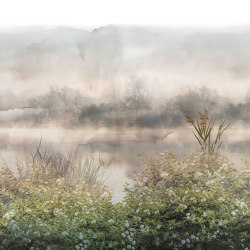This very small square image appears to be an outlined watercolor painting of a hazy, gray, and cloudy landscape. The foreground is dominated by two bushes, each adorned with clusters of small, white flowers concentrated towards the lower half. Alongside these bushes, some taller grasses or shrubs with white blossoms can be noticed, while tiny twigs or branches sporadically poke out. The scene seems to depict a riverbank or pond, extending into the middle ground where more trees and various greenery recede into the hazy backdrop. A wooden structure emerges faintly amidst the blur, suggesting either a distant dock or house. Despite its painterly quality and lack of evident artist initials commonly found in such works, the minuscule size and slight curvature along the top edge make discerning finer details a challenge. The overall impression evokes a serene yet indistinct landscape on a gray, overcast day.